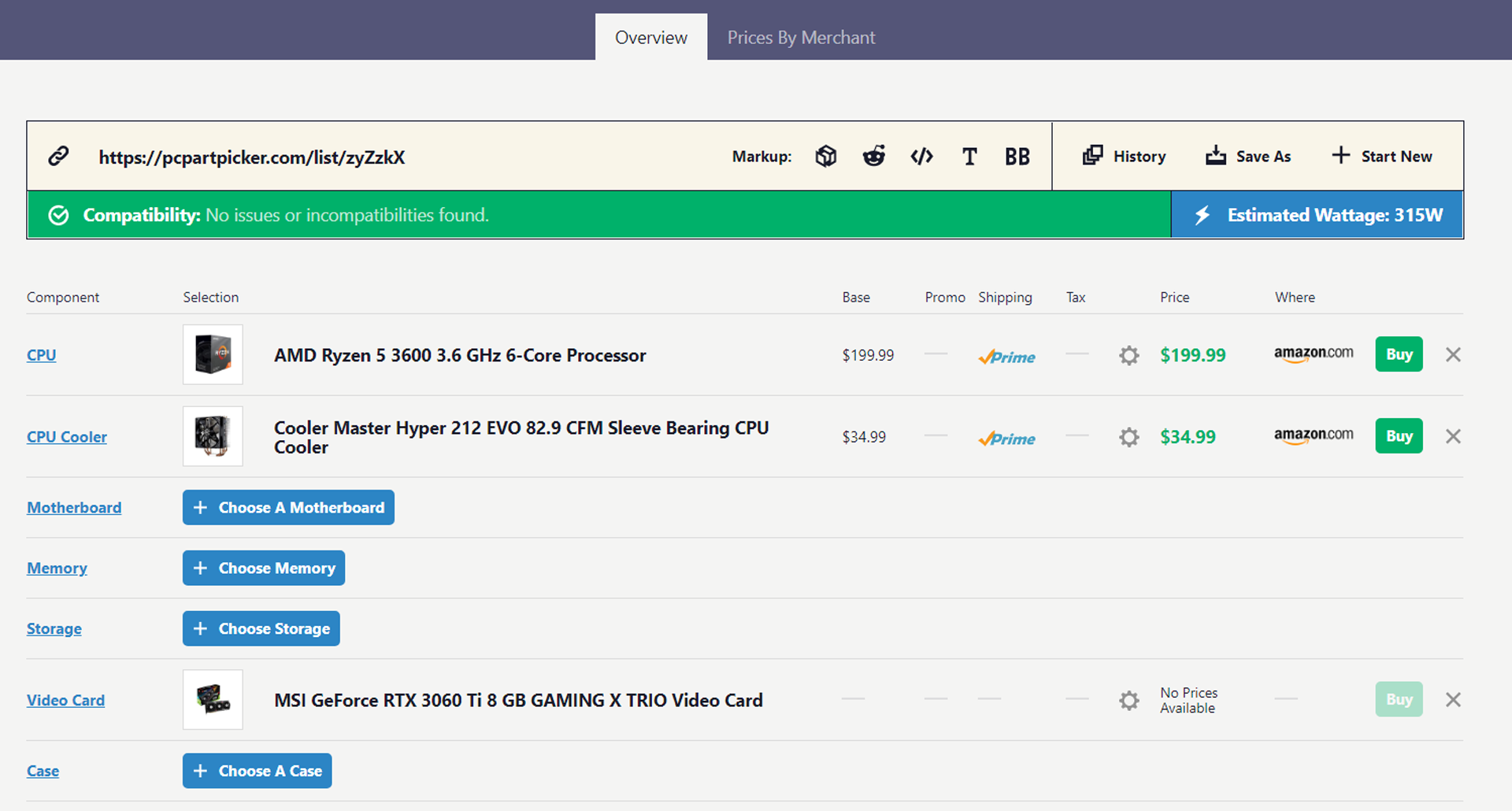This screenshot captures a detailed view of a website with a gray background at the top, featuring a central blue rectangle. At the top, two tabs are present: the left tab is gray with black text reading "Overview," and the right tab matches the blue background color with gray text that says "Prices by Merchant."

Below these tabs, the webpage begins with a beige rectangular section. On the left side of this section, a black paperclip icon is present, followed by the URL "https://pcpartpicker.com/list/ZYZZKX." Further down the same line, "Markup:" is displayed, accompanied by several icons: the Reddit logo, icons for bold and italic text, multiple sheets of paper, a history label, and a notification bell icon. Additionally, the section features a "Save As" label near a plus icon that says "Start New."

The next section contains a green rectangle with white text and a checkmark, stating "Compatibility: No issues or incompatibilities found." Adjacent to this, a blue rectangle with white text indicates "Estimated Wattage: 315W."